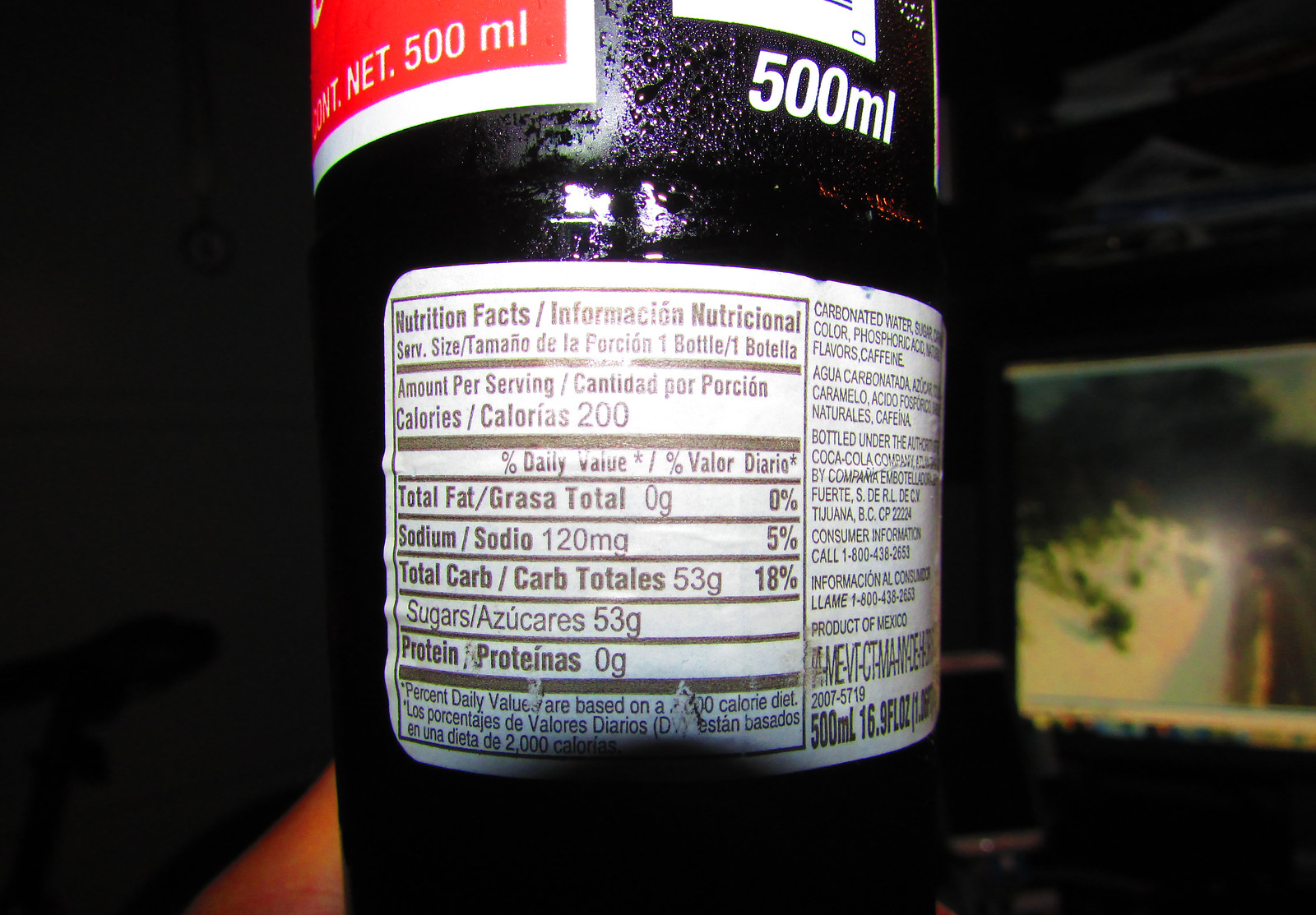The image depicts the back of a sleek, black beverage bottle adorned with a bold red label. Prominently displayed on the bottle in white print is "500 ml," indicating its volume. The focus of the image is the nutritional facts label, although there is a reflective glare making some parts difficult to decipher. Clearly visible on the label are the nutritional breakdowns: total fat is marked at 0 grams, sodium at 120 mg, total carbohydrates at 53 grams, of which sugars also account for 53 grams, and protein at 0 grams. Additionally, the label displays percentage daily values, specifically 0%, 5%, and 18%. Beneath these figures, there is further text too small to be legible in the image.